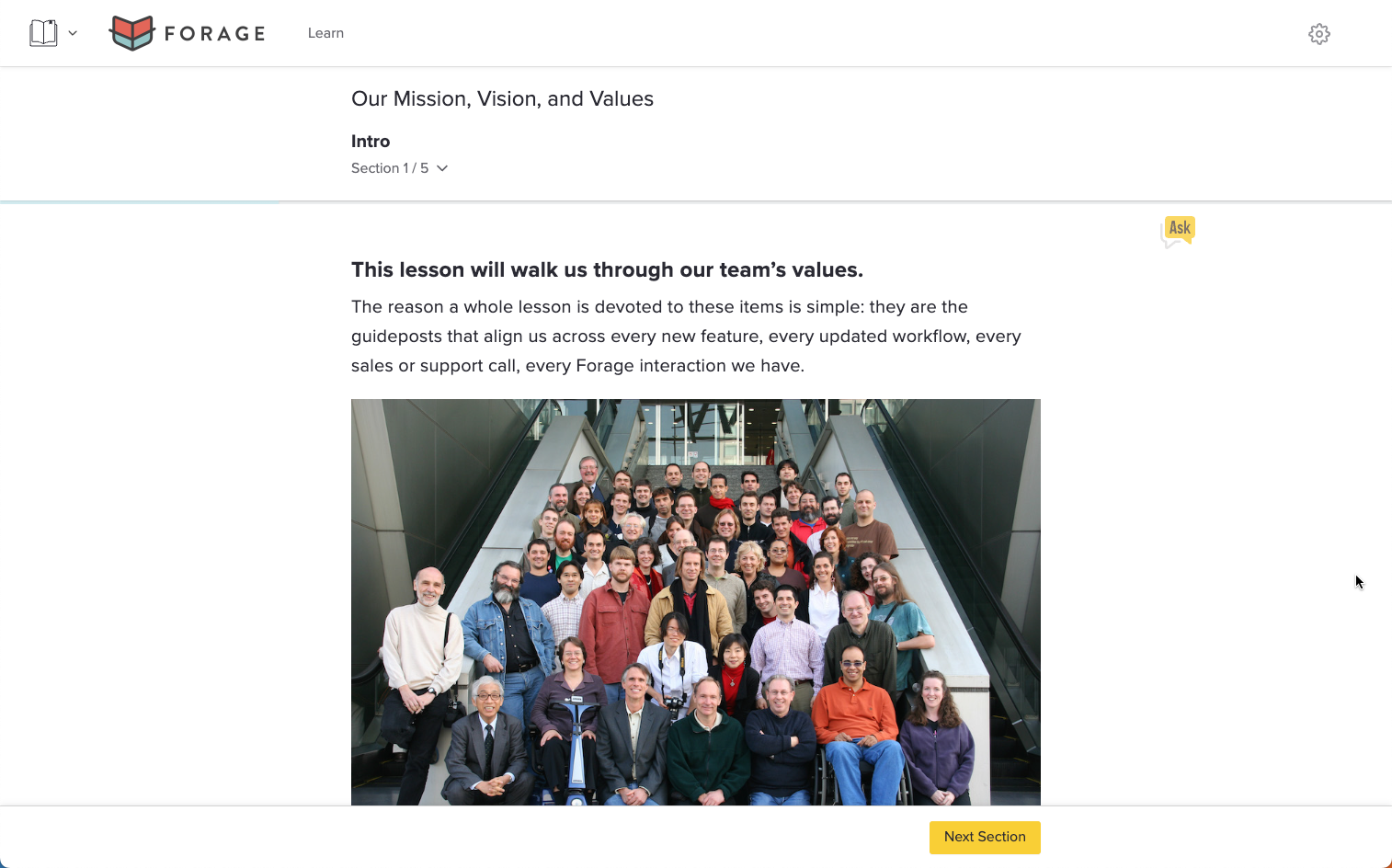Here is a cleaned-up and detailed caption based on the description you provided:

---

This image is a detailed screenshot of the landing page for a company’s website. The page has a clean, white background, illustrating a modern and minimalistic design.

Starting at the top left corner, there is a black line icon of an open book, adjacent to which is the company's logo featuring a stylized arrowhead or feather design, with the top part colored red and the bottom part blue. Next to the logo, the company name "FORAGE" is prominently displayed in bold, black, capital letters. Accompanying this, in smaller, light gray letters in title case, the word "Learn" is positioned to the right of "FORAGE." 

Spanning the top right corner of the page is a settings icon in the form of a cogwheel. Directly below these icons and text elements is a delicate, thin, light gray divider line. Midway on the page, in a centrally-aligned heading, the text "Our Mission, Vision, and Values" is presented in black title case letters, indicating a key section of the webpage. Below this heading, the bold text "Intro" is followed in light gray, thin letters by "Section 1 of 5" with an arrow pointing downward.

Another thin, gray divider line follows before the main content section. The central focus of this area begins with the bold text "This lesson will walk us through our team's values," expressing the introductory overview. Adjacent to this text, located in the upper-right corner of the section, is an interactive icon resembling a yellow and white chat bubble with the word "Ask" inscribed in black letters.

Further down, the main body text elaborates, "The reason a whole lesson is devoted to these items is simple. They are the guide points that align us across every new feature, every updated workflow, every sales or support call, every Forge interaction we have." This paragraph underscores the importance of the company’s guiding principles.

Below this detailed explanation is a photograph depicting the company’s team, approximately 50 members, arranged on a wide, modern staircase within a spacious, corporate building. The team members are positioned in seven approximate columns, though they are staggered in various rows, with some kneeling or sitting in the front.

At the bottom right of the page, there is a prominent yellow button labeled "Next Section," inviting the user to proceed to the following part of the website.

---